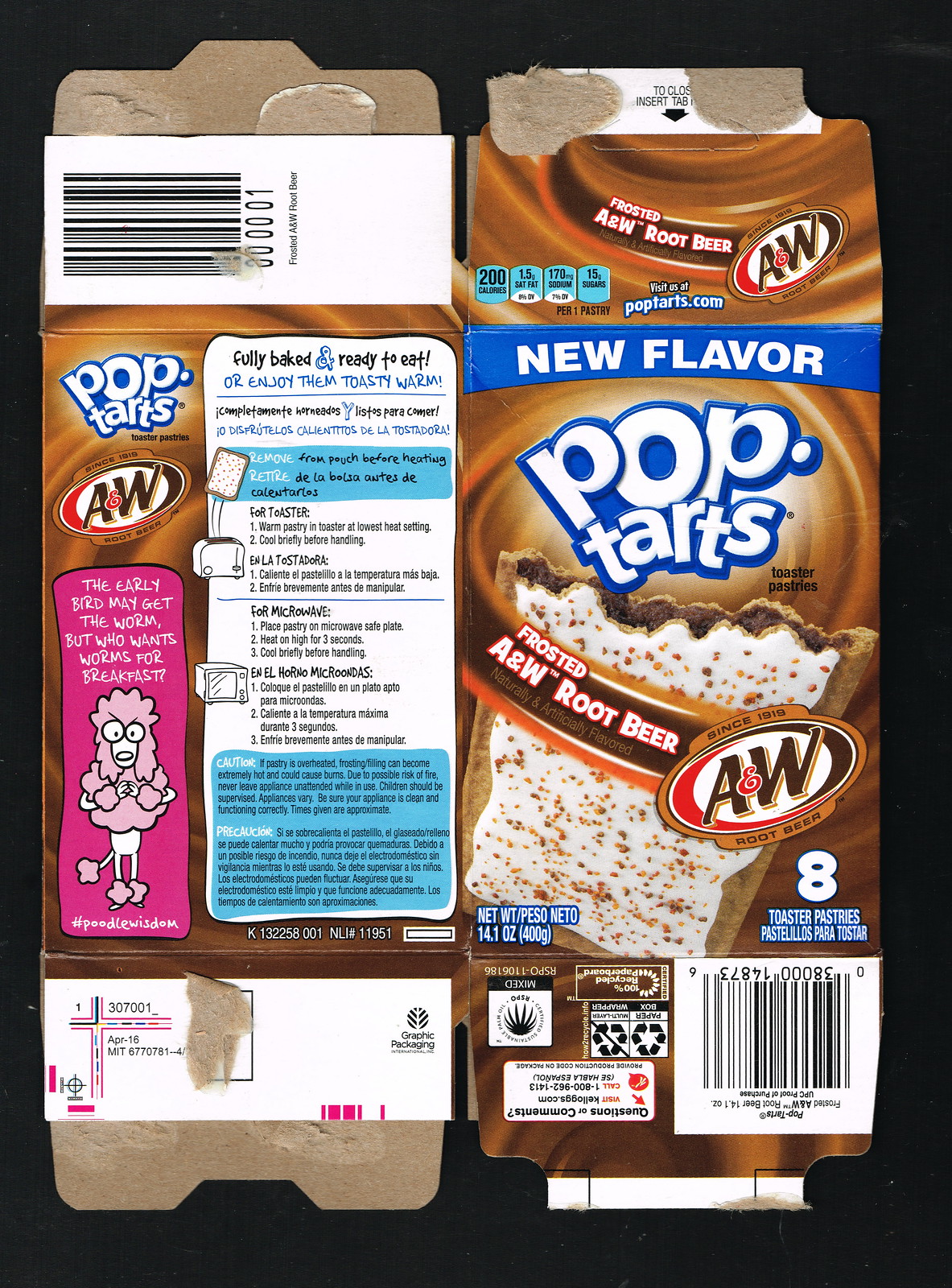This image depicts a fully flattened Pop-Tart box, prepared for recycling. The black background accentuates the box, allowing for a clear view of both its front and back labels. The front prominently advertises a unique, new flavor: Frosted A&W Root Beer, featuring a visual of a white-frosted Pop-Tart filled with a dark filling. The packaging details that the box contains eight toaster pastries, weighing a total of 14.1 ounces.

The back of the box offers a whimsical touch, with text proclaiming, "Fully baked, ready to eat or enjoy them toasty warm. The early bird may get the worm, but who wants worms for breakfast?" Accompanying this playful statement is a colorful cartoon illustration of a pink and white poodle, under the banner of "#PoodleWisdom." The overall design blends humor and nostalgia, enticing both Pop-Tart enthusiasts and curious snackers alike.